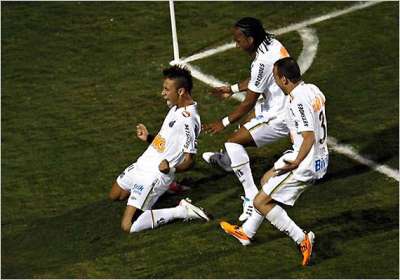In this dynamic image set on a dark green soccer field, three darker-skinned athletes dressed in matching white uniforms with orange accents and assorted sponsorship insignias are captured in a jubilant celebration. The field, partially visible with cream-colored lining and a circular mark at the corner, indicates this might be near the goal area. The lighting suggests it was taken in the later part of the day or possibly in the evening.

The central figure, a man with black short hair, kneels on the ground with fists clenched at his sides, his face lit up in a triumphant yell, possibly celebrating a goal. His visible excitement is met by his two teammates approaching from behind. To his left, one teammate with wristbands is crouched, seemingly ready to support or embrace the central figure, while the third teammate, wearing orange cleats and with the number three visible on his uniform, approaches from the right. His side profile shows off long black dreadlocks.

This image powerfully captures the moment of victory and the collective emotion between the players, united in their shared success on the field.